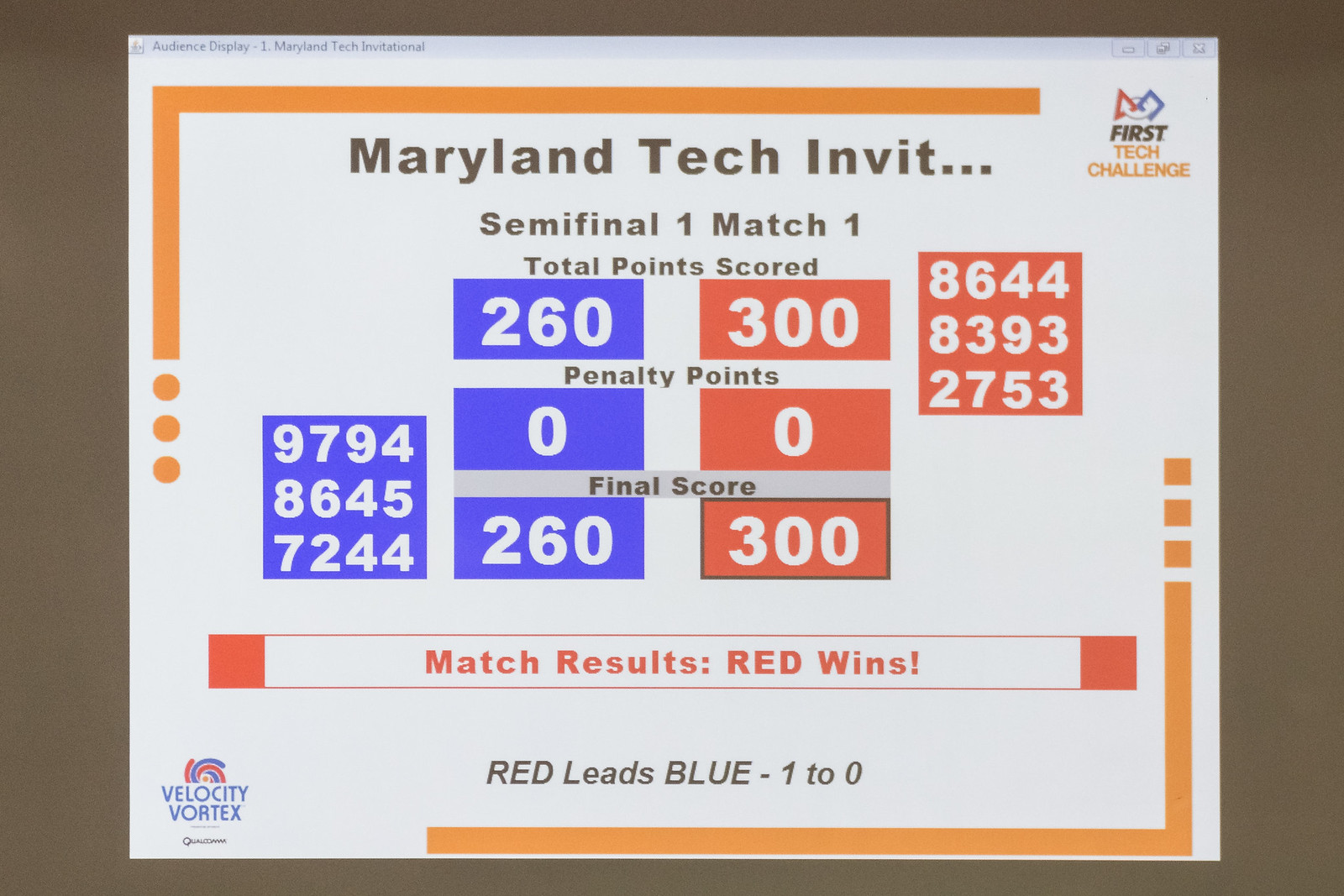The image is of a presentation slide resembling a scoreboard, bordered with an orange frame featuring circles and red squares. The header reads "Maryland Tech Invitation" with the subheading "Semi-Final 1, Match 1." The slide is divided into two sections: the left section is blue and the right section is red. The content reads as follows: 

Total point score: Blue – 260, Red – 300.
Penalty points: Blue – 0, Red – 0.
Final score: Blue – 260, Red – 300.

The match results in red writing state: "Red wins," and in black writing underneath, it reads: "Red leads Blue 1-0." The slide appears to be a projection or a computer window against a grayish background.